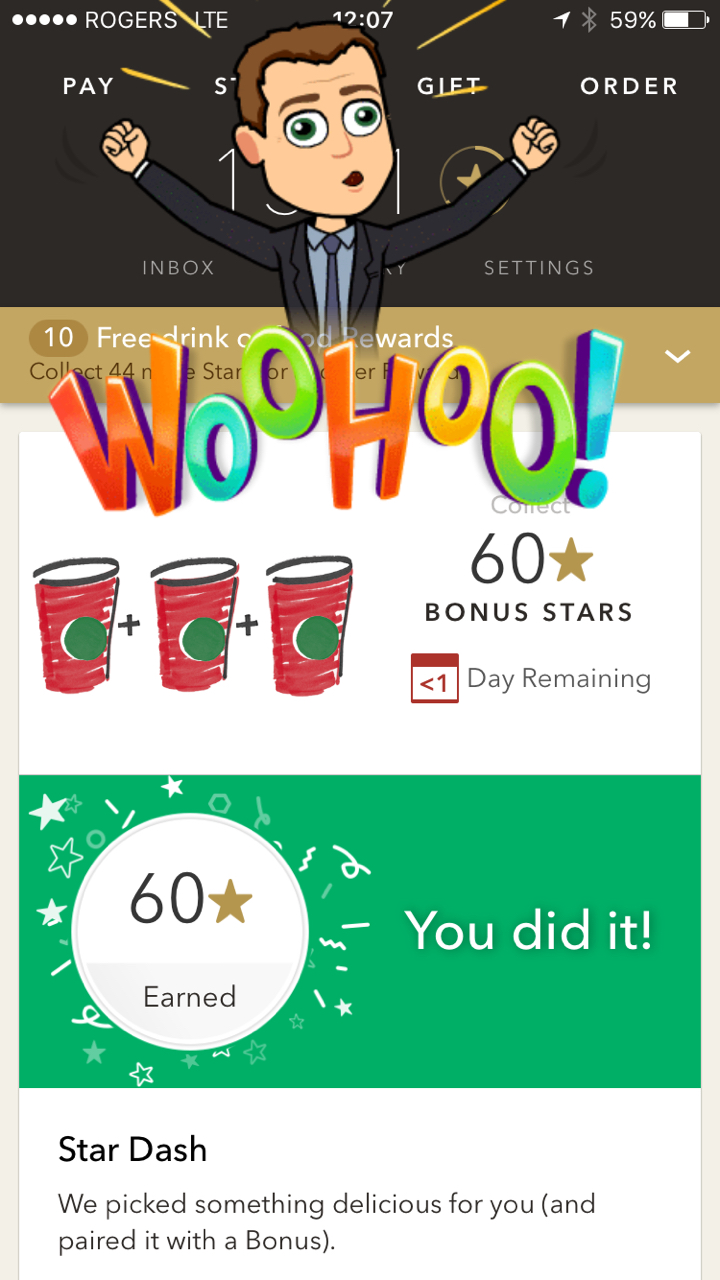The image is a screenshot from a mobile app captured on a cell phone. At the top left corner, it says "Rogers LTE," and to the right, it shows a translucent gray Bluetooth icon and indicates the battery life at 59%. The time is displayed in the center as "12:07," though it does not specify AM or PM. The main section of the screen features a colorful cartoon figure of a man with brown hair, wearing a suit and tie, with both arms raised in the air. Above him, "Woohoo!" is written in vibrant, rainbow-colored letters. Below him, there are three rough-sketch style coffee cups with plus signs between them, alongside a gold star symbol and text stating "60 bonus stars." Additionally, there's a small calendar icon indicating "1 day remaining." At the bottom, a green horizontal stripe reads "60 stars earned. You did it!" Further down, on a white panel, it says, "Star dash: We picked something delicious for you and paired it with a bonus."